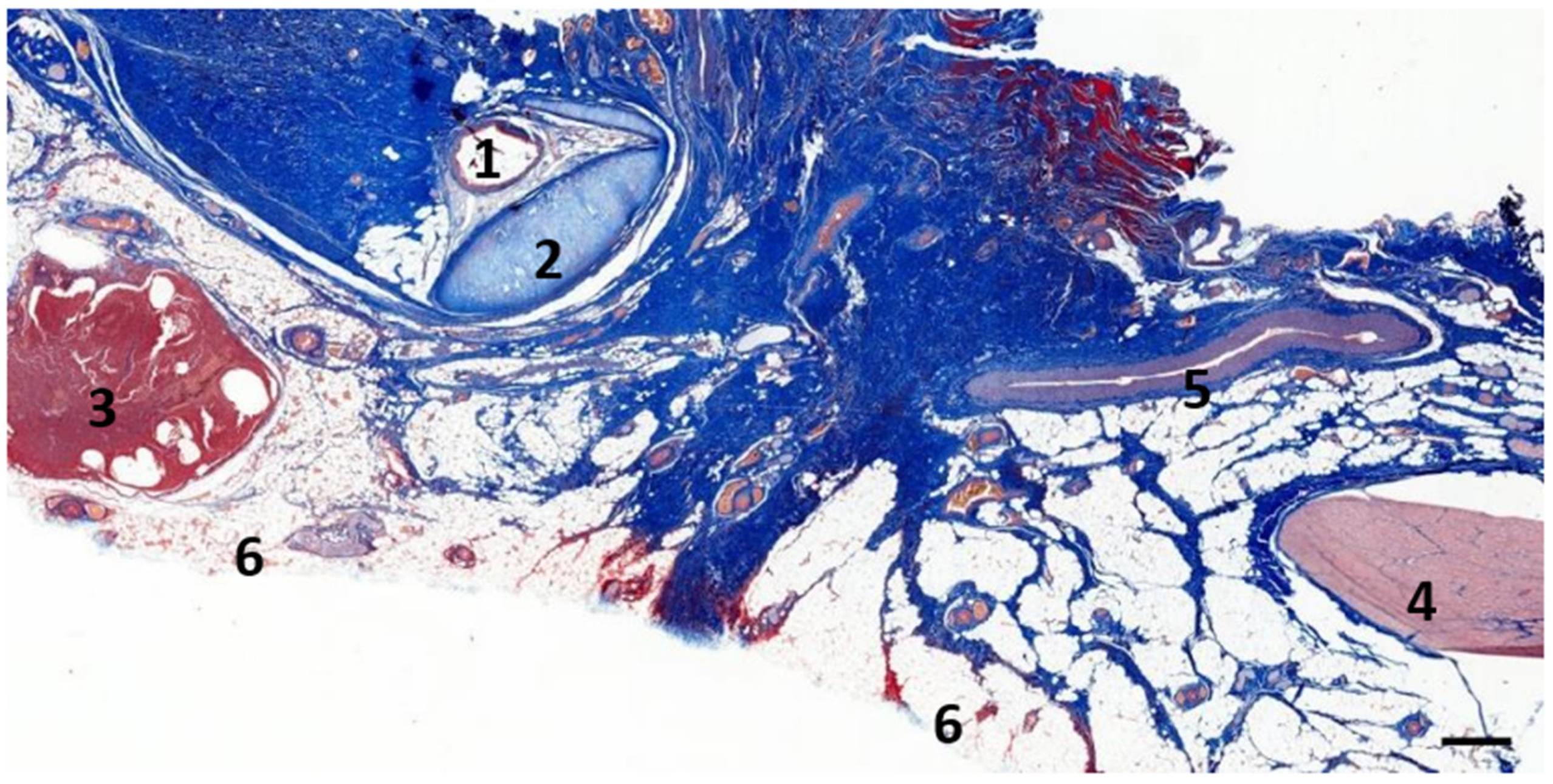The image is a detailed and colorful diagram, which appears to be a highly magnified view of either a biological cell or possibly an abstract representation of geographical features like land masses and water. The dominant color in the diagram is royal blue, which extends from the top left toward the lower right, covering the majority of the image. This blue area contains a white circle labeled "1." Directly below this circle is a lighter blue, almond-shaped region, outlined in royal blue and labeled "2."

To the left of these blue areas, there's a red blob-like section with patches of white, labeled "3." On the far right side of the image, another almond-shaped area can be seen, this time in pink, labeled "4." Above this pink section is a long, thin white swirl with a small red and white bulb on its end, which is labeled "5."

The diagram also has several other colors splattered across it, including shades of red, light blue, and a peachy-pink hue. A small black line is located on the lower right side of the image. The number six appears twice within the whitish regions that border and intersperse the various colored sections.

Each numbered section represents different areas, suggesting a complex and layered structure. The repeated number six on whitish areas hints at recurring elements or significant border regions that frame the diagram's primary features.